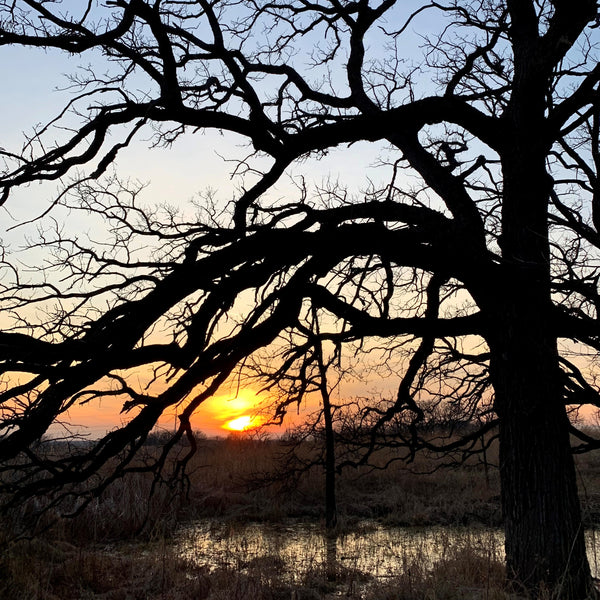This square outdoor photograph, approximately four inches by four inches, captures a serene and detailed landscape during daytime. Dominating the right side of the image, a large, black-shadowed tree stands tall with its wide trunk extending from the bottom to the top of the frame. Its branches fan out towards both sides, with some reaching across the left side of the picture and even out of the frame. Beneath the tree lies a small, dark, swampy pond reflected in still water, bordered by tall grasses. The background reveals a gradient sky, transitioning from an orange and peach near the bright white and yellow sun, which is partially obscured by clouds, to a light blue and finally a deeper blue at the top. This captivating backdrop is completed with a field of lush grass behind the water, adding to the tranquility and depth of the scene.